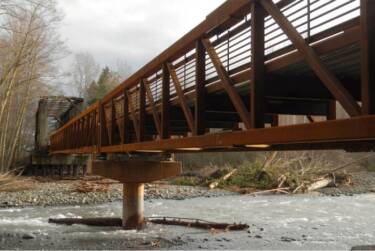In a square, full-color photograph taken during daytime in either fall or winter, we see a prominent rusted, brown metal bridge featuring an N-shaped pattern across its sides and crisscrossing girders for support. Below the bridge flows a greyish-white river, dotted with stones and debris, with visible support beams plunging into the water. On the near bank of the river lie grasses and numerous grey stones, alongside downed tree trunks. To the left of the image, leafless, tall, and skinny trees stand, contributing to the stark, wintry atmosphere. In the background, the bridge arches over a short, darker brown tunnel, adding depth to the scene, with a sky hovering above and hinting at the seasonal chill. The image excludes any signs of people, animals, or text.